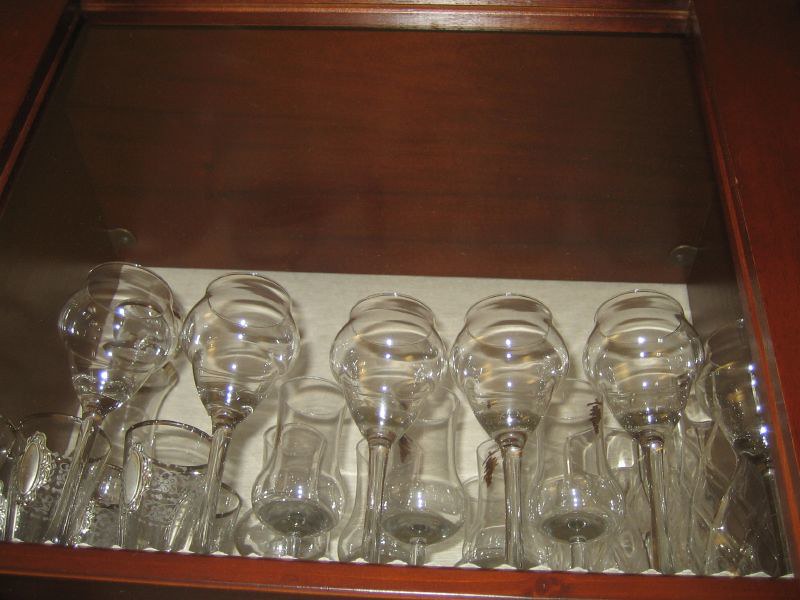Inside a mahogany-colored wooden cabinet with a glass front, a variety of crystal-clear glassware is neatly arranged. In the front row, there are several elegant wine glasses, each with long stems and flower-shaped bulbs that suggest occasional, fancy use. Directly behind these are clear drinking glasses adorned with intricate silver medallions, rims, and embossing, adding a touch of sophistication. To the right, several large goblets with short stems and wide, flared bowls are positioned, while a distinctive pitcher with a cross-hatched design stands at the far end. The glassware appears clean and meticulously displayed, reflecting light from the glass backing and creating a sense of depth within the cabinet. The arrangement suggests that these pieces are cherished and likely reserved for special occasions, with the cabinet itself serving as both a functional storage piece and a showcase for these refined items.